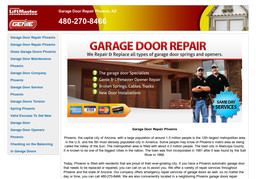The webpage is somewhat small and of low resolution, making its text hard to read. At the top, there is a reddish-orange banner with white text in the top left corner, which is difficult to decipher due to its small size. Prominently on the page is a headline in large red capital letters reading "GARAGE DOOR REPAIR." Below this, in gray text, it states, "We repair and replace all types of garage door springs." The banner on the top contains a small picture of a white house with two garage doors.

On the left side of the webpage, there's a long list of about 15 blue links. Directly below the headline "GARAGE DOOR REPAIR," there's an image showing the exterior of a house with two brown garage doors. To the right of the image are two individuals dressed in black shirts. Additionally, a blue area on the image reads "Same-Day Services," while an orange section on the left lists accepted payment methods, including Visa and MasterCard. Underneath this area is a black headline followed by two paragraphs of black text.